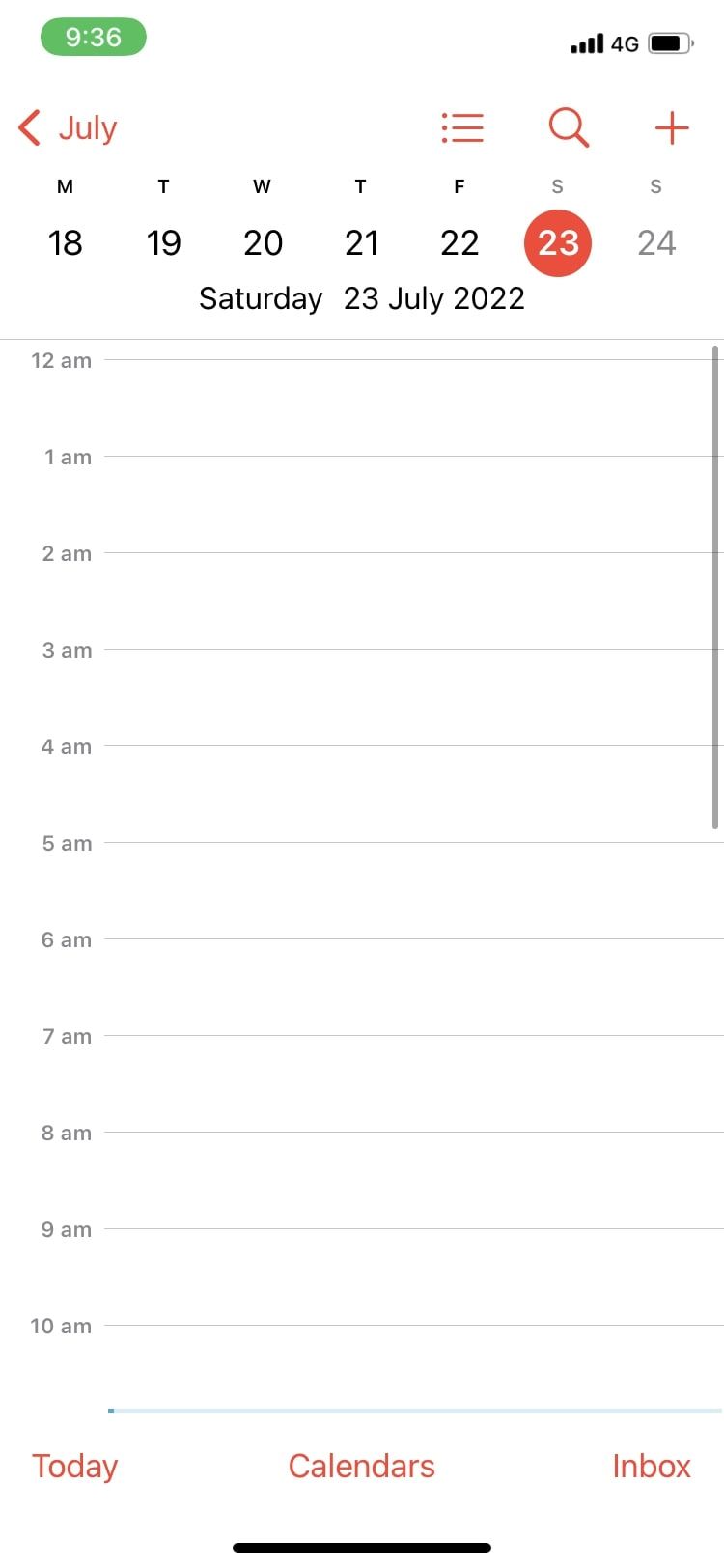The upper left corner of the white background features a green oval with "9:36" displayed in white text. On the right, there are four black bars indicating full service, accompanied by a "4G" symbol in black and a battery icon showing approximately 85% charge. 

On the left side, in red, there's the end of an arrow pointing left, followed by the word "July" with a capital J. Below this, there are three red circles with horizontal lines, a red magnifying glass, and a red plus sign. 

Directly beneath, the days of the week are listed, with "M-T-W-T-F" in black and "S" in grey, despite Sunday traditionally being the first day of the week. 

Underneath the days, the numbers 18 through 22 are displayed in black. The number 23 is highlighted in white with a red circle around it, and the number 24 is shown in green. 

Below these numbers, "Saturday, 23rd of July, 2022" is written in black text, followed by a timeline marked in grey from 12 a.m. to 10 a.m. 

At the bottom, in red, the words "Today," "Calendars," and "Box" are visible.